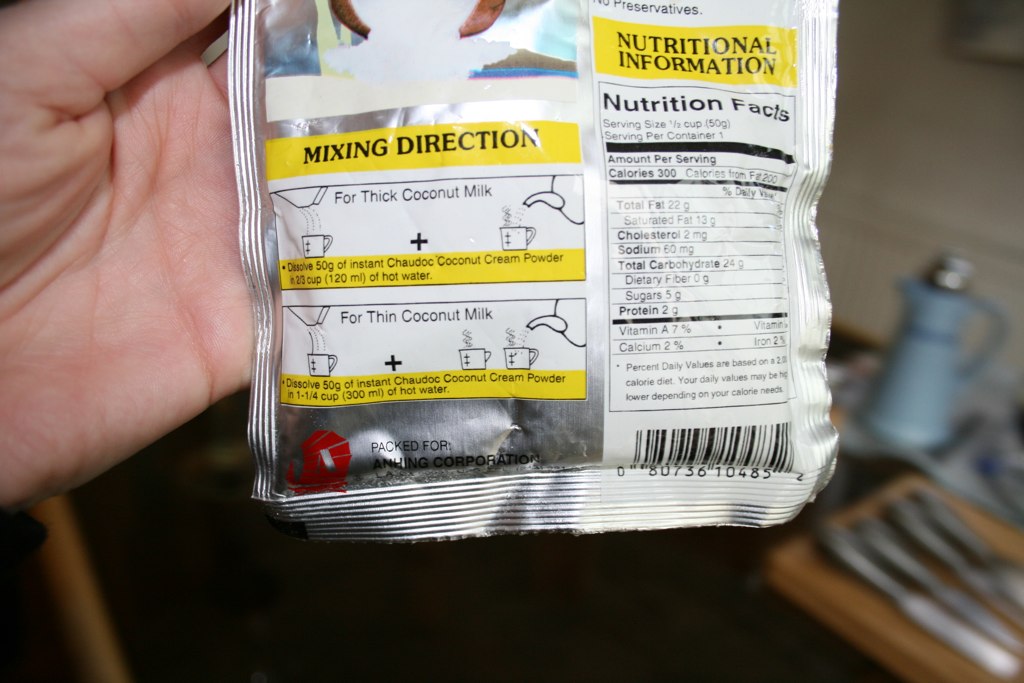In the image, a person is holding out their hand, while at the very top left corner, there's a clear picture. An open coconut is visible, pouring out what appears to be coconut milk. On the left side of the image, a yellow rectangle contains detailed nutritional information including serving size, calories, and nutritional values for various components such as total fat, saturated fat, and protein. Below this, another yellow rectangle provides mixing directions in black text. It instructs to dissolve 500 grams of instant chocolate coconut cream powder for a thick coconut milk consistency and continues with directions for making a thinner version. There are two mugs visible on the right side and a mug on the left, suggesting the mixture is being poured into these containers. The bottom of the image features some silver elements, possibly a reflective surface.